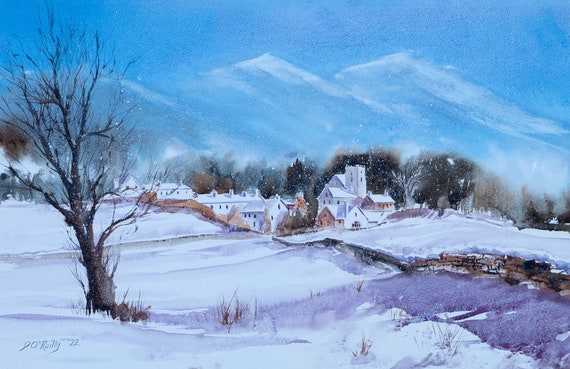The image appears to be a detailed painting of a serene winter landscape. Dominating the scene is a snowy field that stretches from the foreground to a charming town in the distance, dotted with white and beige buildings. On the bottom left corner of the painting, there is a barren tree with three major branches, positioned prominently. A delicate signature, possibly reading "D’O’Rolly 22," is also discernible there, though the writing is light and small. 

A stone wall, subtly covered in snow, runs diagonally across the center of the image. This divides the snowy foreground, where patches of brown grass peek through the snow, from the town that lies nestled in a slight valley. Behind the town, a thicket of trees, depicted in shades of black and brown, extends horizontally and seems almost to blend into the sky. 

In the backdrop, a range of large, white mountains looms majestically, creating a striking contrast with the bright blue sky above them. To the right of the town, greyish patches, possibly representing snow-covered plants, add to the layered complexity of the scene. The entire setting is rendered in bright and clear lighting, bringing vibrancy and depth to the tranquil winter landscape.